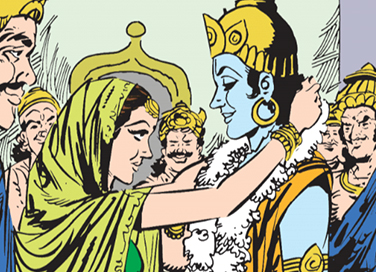In this detailed full-color cartoon illustration, likely created digitally, the scene appears to be inspired by Middle Eastern or Indian cultural themes and may derive from a comic book aesthetic. The artwork is presented in a square format without a distinct background, except for a large white column-like building with a yellow arched doorway that subtly anchors the setting. The focal point of the image is a solemn interaction between a woman and a blue-skinned man who exudes a deity-like presence. The woman, who has dark hair, is adorned in a green dress with a yellow-green shawl that covers her head and shoulders, and she is placing a white flower lei around the man’s neck. Her head is slightly bowed in reverence, yet she gazes up at the man through lowered lashes. This man is characterized by his striking blue skin, black hair, a large gold hoop earring, a gold hat, and a gold band on his bicep. Surrounding the central figures are five men, each wearing gold helmets and blue or toga-like outfits. These onlookers exhibit various mustachioed expressions, adding to the theatrical and reverent ambiance of the scene, as they observe the ceremonial act taking place.